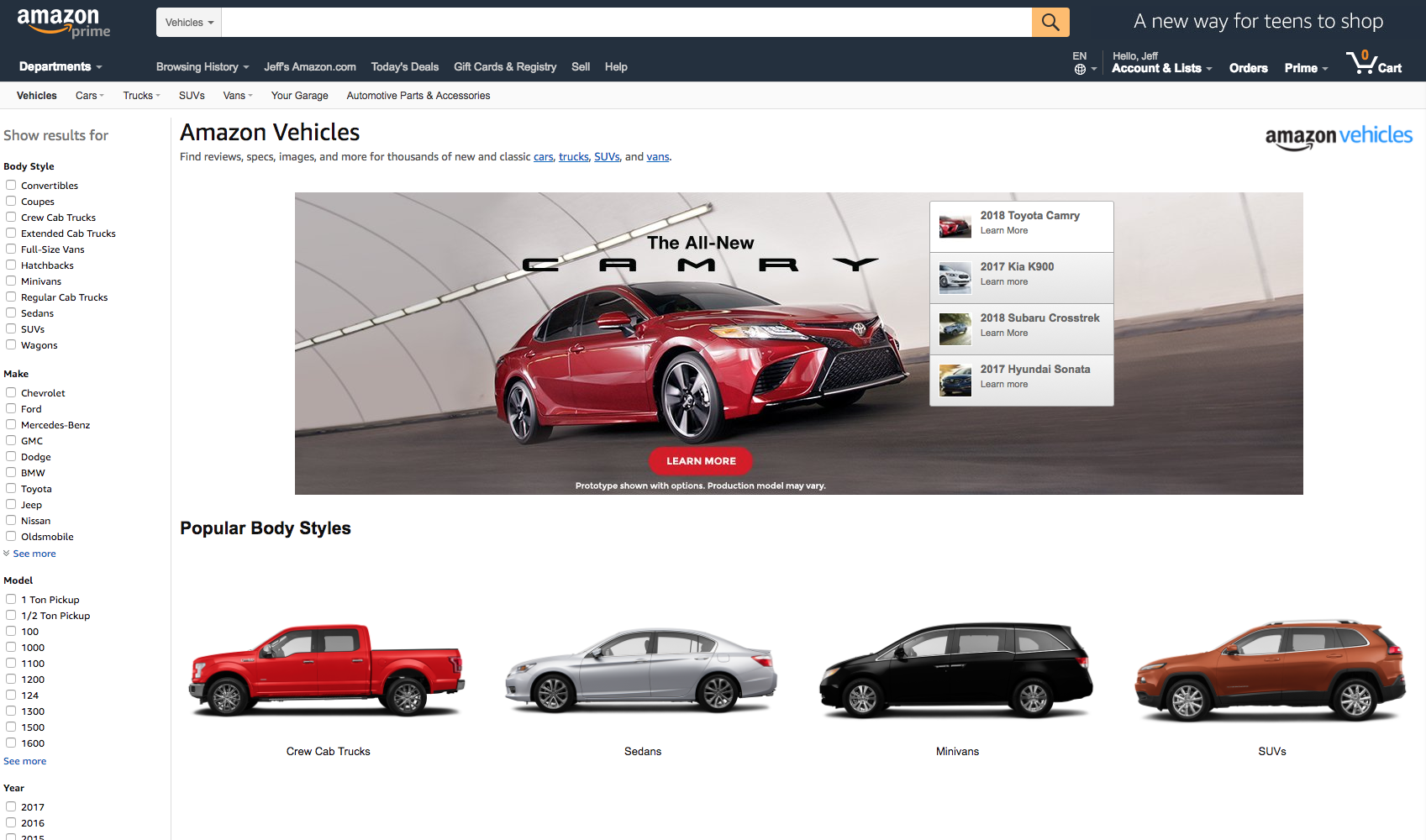This is a detailed screenshot of the Amazon Vehicles webpage. At the very top, the Amazon Prime banner prominently appears alongside the search bar. Below this, within the Amazon Vehicles section, the featured ad highlights reviews, specifications, images, and additional vehicle suggestions. The centerpiece of the page is a high-resolution color photograph of a striking red Toyota Camry, occupying almost half the screen. Above this image, a red button invites users to "Learn More" about the vehicle.

On the right, a suggestion box offers related vehicle recommendations, tailored to the interests of someone viewing the Camry. The listed recommendations include a 2018 Toyota Camry, along with models from Kia, Subaru, and Hyundai. At the bottom section, there are thumbnail images of four additional vehicles, all oriented to face left. These vehicles include a red crew cab truck, a silver sedan, a black minivan, and a small rust-colored SUV.

To the left side of the screen, a detailed list of search filters is provided. These filters allow users to narrow down their search based on body style, make, model, and year, enhancing the user experience on the Amazon Vehicles platform.